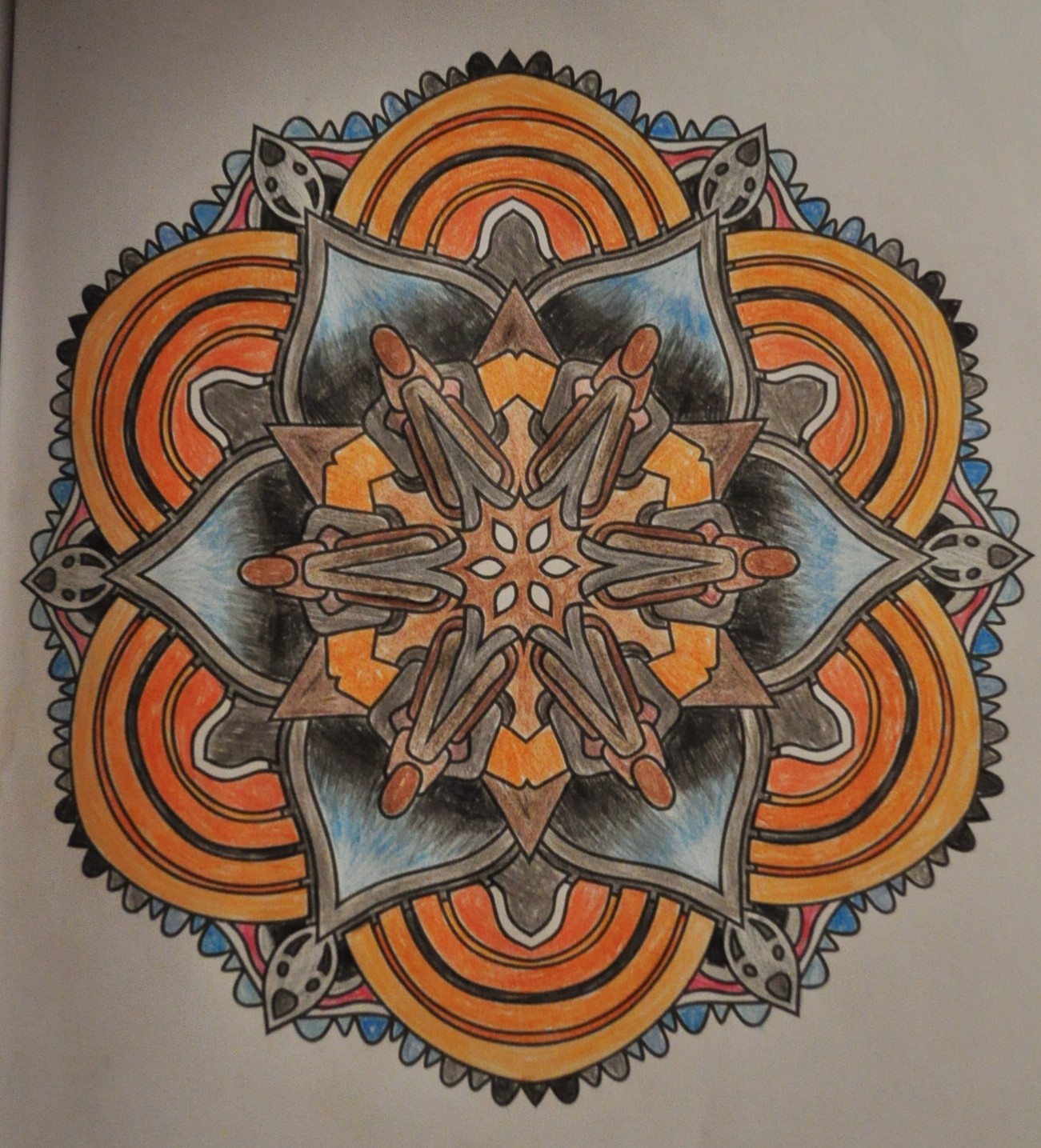The drawing features an intricate and surreal flower with multiple detailed components. The flower's center displays a complex combination of colors and shapes, starting with a small spiky orange ball adorned with six tiny white, apple seed-like elements. Surrounding this are orange spikes arranged in a star shape, adding to the central intricacy. 

Moving outward, the flower features a sequence of concentric rings in varying colors: orange, red, orange, black, orange, light orange, and finally orange again, with a crisp white at the outer rim of this arrangement. Importantly, the structure of these rings isn't circular but rather points, reminiscent of spearheads, colored in shades of gray and light gray.

Between the orange rings, there are peculiar gray "mouth" shapes that add an unusual characteristic to the design. The flower itself is encased in blue, tooth-like structures that form the outermost boundary.

The overall composition of the flower merges natural floral aesthetics with abstract, geometric, and slightly surreal elements, rendering an artwork that is both detailed and captivating.